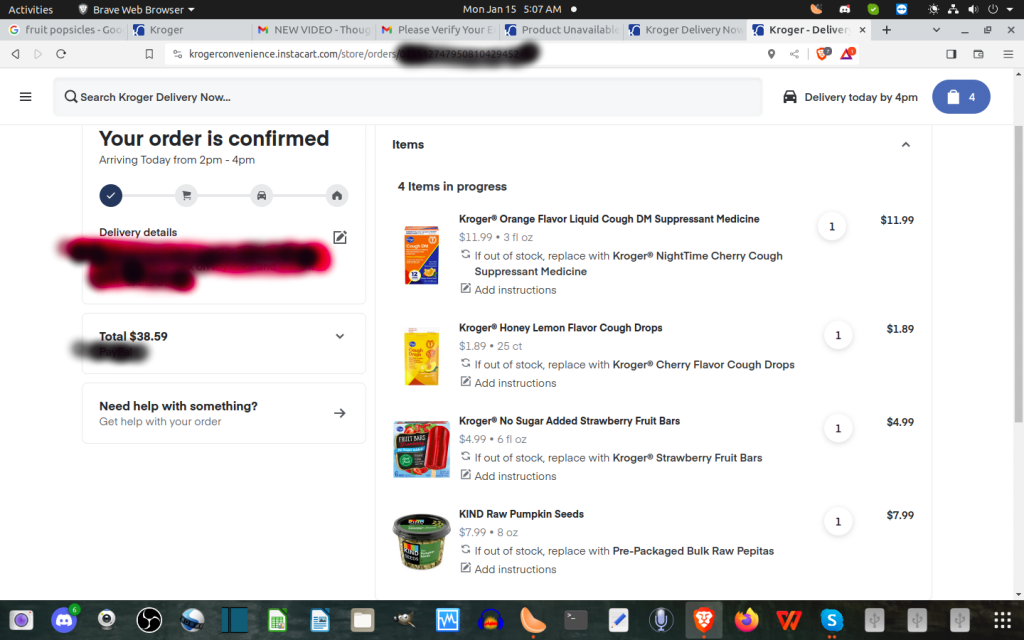A detailed screenshot from a computer shows multiple browser tabs open, with the current tab highlighting an "Order Confirmed" page for an online grocery purchase. The order contains four items in progress: Orange Flavored Cough Syrup priced at $11.99, Cracker Honey Lemon Flavored Cough Drops for $1.89, No Sugar Added Strawberry Fruit Bars at $4.99, and Pumpkin Seeds costing $7.99. The total amount for the order, $38.59, is somewhat highlighted but obscured by red markings. Below this total, additional details about the delivery are indicated, specifying that the items are scheduled to arrive today between 2 to 4 PM. The page also features several icons corresponding to the items listed.